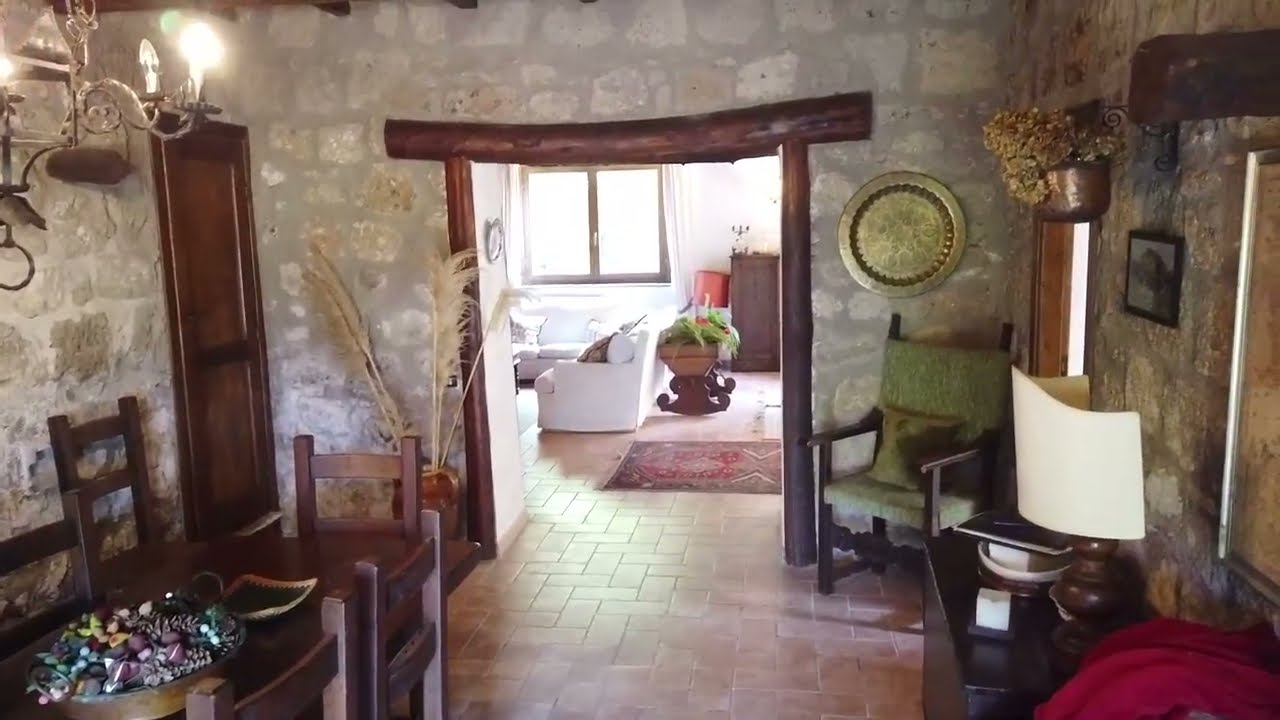The image is a rectangular photograph showcasing the interior of a historical stone house, highlighted by its rustic and primitive decor. The focal point is a kitchen or dining area with a dark brown wooden rectangular table on the bottom left, surrounded by matching chairs. A silver vintage chandelier hangs above the table, which has an oval centerpiece filled with flowers, pine cones, and potpourri. Adjacent to the table, against the gray stone wall, stands a buffet-type piece of furniture with a wooden lamp that has a white lampshade and a black-framed black-and-white picture behind it.

In the right-hand corner, a green and brown vintage chair is situated below a large bronze medallion hanging on the wall. Nearby, a metal pot with dried flowers is positioned above the lamp. The walls, composed of large fitted stones with dark gray mortar, contribute to the historic ambiance, complemented by dark stained wooden trim and beams.

A prominent rectangular doorway made of dark brown logs grants a view into the adjoining room. This adjacent space features a white couch, a planter with ferns in a cradle-like dark wood base, and a Persian-style rug on the floor. A large window with two openings and a clock on the left-hand wall are also visible. The consistent primitive wood and stone theme extends into this next room, maintaining the cohesive historic aesthetic.